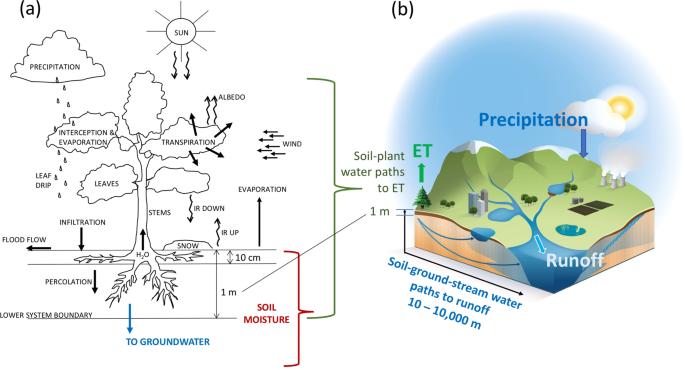This infographic, divided into two sections labeled A and B, comprehensively illustrates the water cycle and its impact on the environment. 

On the left side (A), depicted in a detailed black and white line drawing, a tree stands at the center with various natural and hydrological processes labeled around it. These labels include "Sun," "Precipitation," "Interception," "Evaporation," and "Transpiration" among others, with arrows pointing to relevant parts of the tree, ground, and sky. The tree's root system is shown penetrating about a meter into the ground, where processes such as "Percolation" and "Infiltration" are illustrated. The drawing also includes terms like "Flood Flow," "Stem," "Snow," "H2O," and "Lower System Boundaries to Groundwater." Text in red and blue colors highlight areas like "Soil Moisture" and "Groundwater," signifying key components of the water cycle.

On the right side (B), a colored digital illustration complements the information in A by depicting a broader landscape. This section showcases a mountainous region with a lake, city, trees, and a power plant under the sun and clouds. It uses color to differentiate elements and processes such as "Precipitation" from clouds and "Runoff" into rivers and lakes. This graphic emphasizes the journey of water from precipitation to various water systems, with terms like "Soil," "Ground Stream Water," and the range "10 to 10,000 meters" indicating the scale of water movement through the environment.

Together, these sections illustrate the comprehensive flow of water from precipitation to its absorption and movement through plants and soil, providing a multi-faceted view of the hydrological cycle.